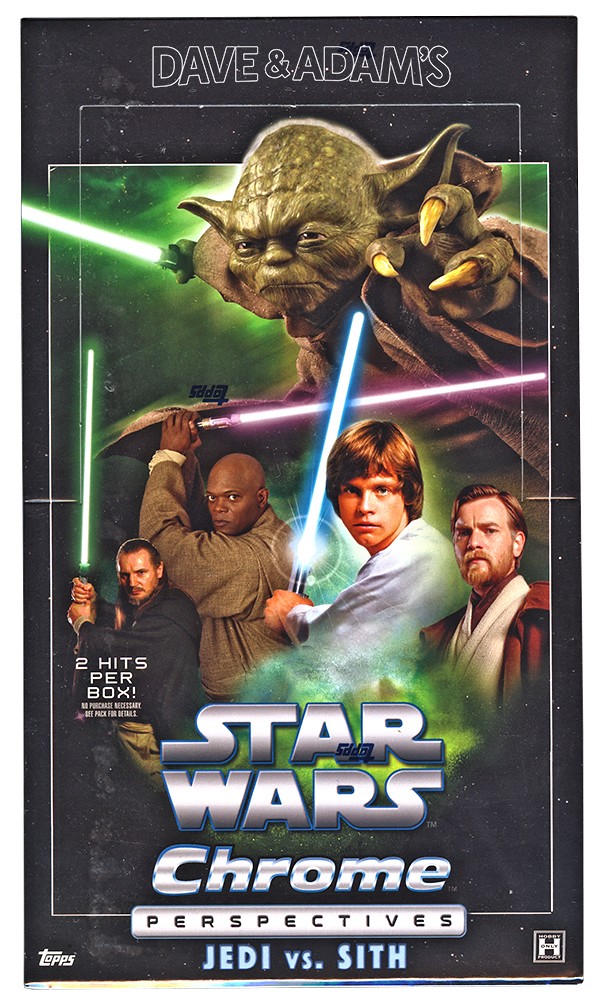The poster advertising Star Wars has a striking black background resembling a night sky filled with white stars. At the top of the poster, in black text with a white outline, the names "Dave and Adams" are prominently displayed, surrounded by some white squares. Right above the center, a dynamic image of Yoda is shown leaning forward with his one hand extended, revealing long yellow claws, and his other hand gripping a green lightsaber. Below Yoda, four distinct characters from the Star Wars universe are depicted: on the far right, a young Ewan McGregor as Obi-Wan Kenobi, clad in a white and amber-colored robe; next to him, Mark Hamill as Luke Skywalker holding a blue lightsaber pointed upwards and to the right; beside him, Samuel L. Jackson brandishing a purple lightsaber above his head; and to the far left, Liam Neeson with a green lightsaber. Underneath Neeson's image, the text "two hits per box" is written in small print. Directly beneath Luke Skywalker, the title "Star Wars Chrome Perspectives: Jedi vs Sith" is featured prominently. The bottom corners of the poster include the "Topps" logo on the left and a square with the letter "H" inside it on the right. The entire image is outlined with a continuous white line, framing the characters and text.